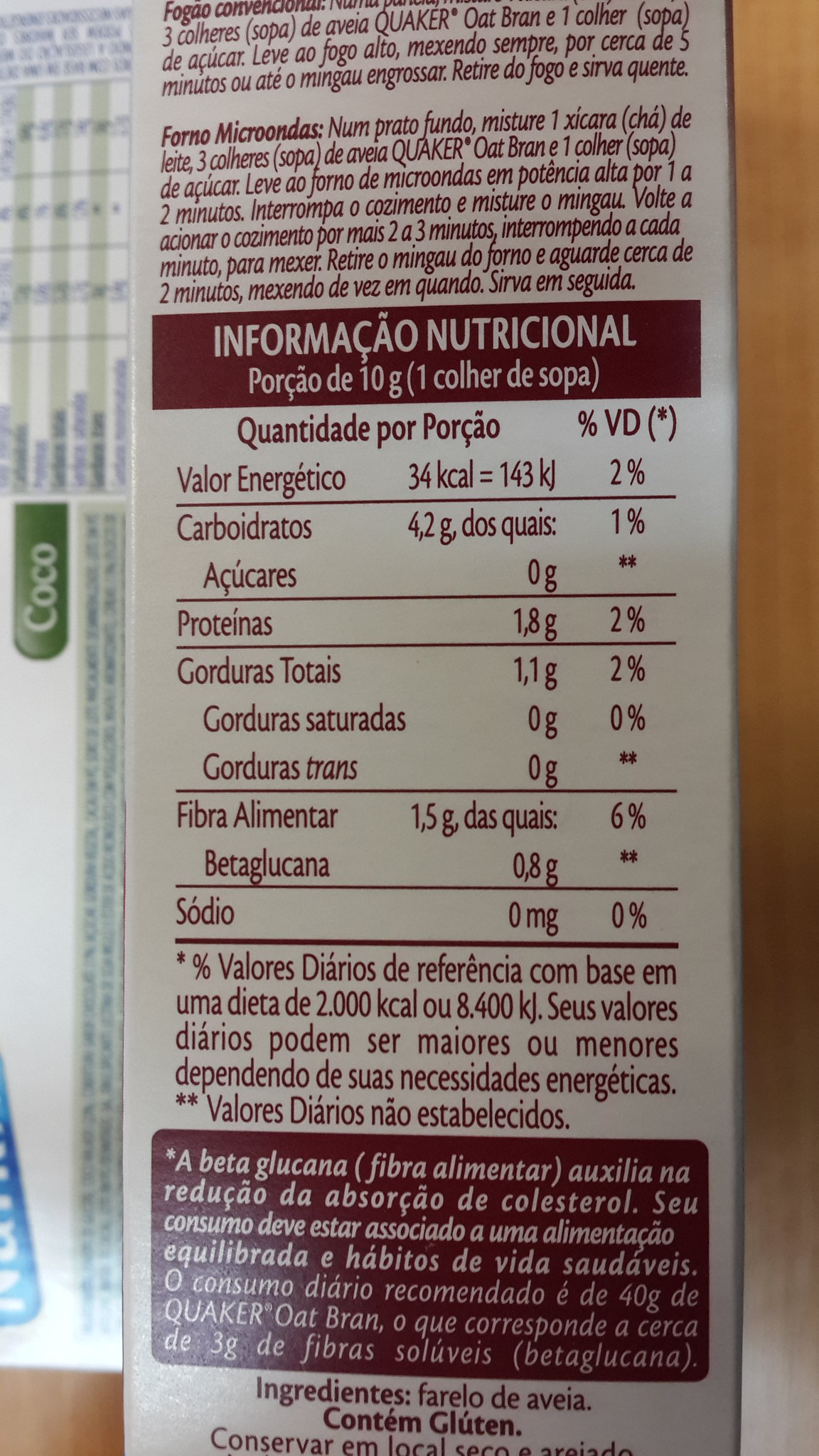This photograph captures a close-up of the nutrition label on the side of a white Quaker Oat Bran food container, featuring red text predominantly written in Spanish. The label provides detailed nutritional information, including amounts per serving: 4.2 grams of carbohydrates, 1.8 grams of protein, 1.5 grams of fiber, and 0 milligrams of sodium, delivering 34 kcal of energy per serving. Positioned on the left side is a small green box with the word "Cocoa" printed in white letters. The background to the right features a strip that reveals a wooden tabletop. The overall setting and informational content suggest a focus on the product's dietary specifications, though some of the finer prints are illegible.